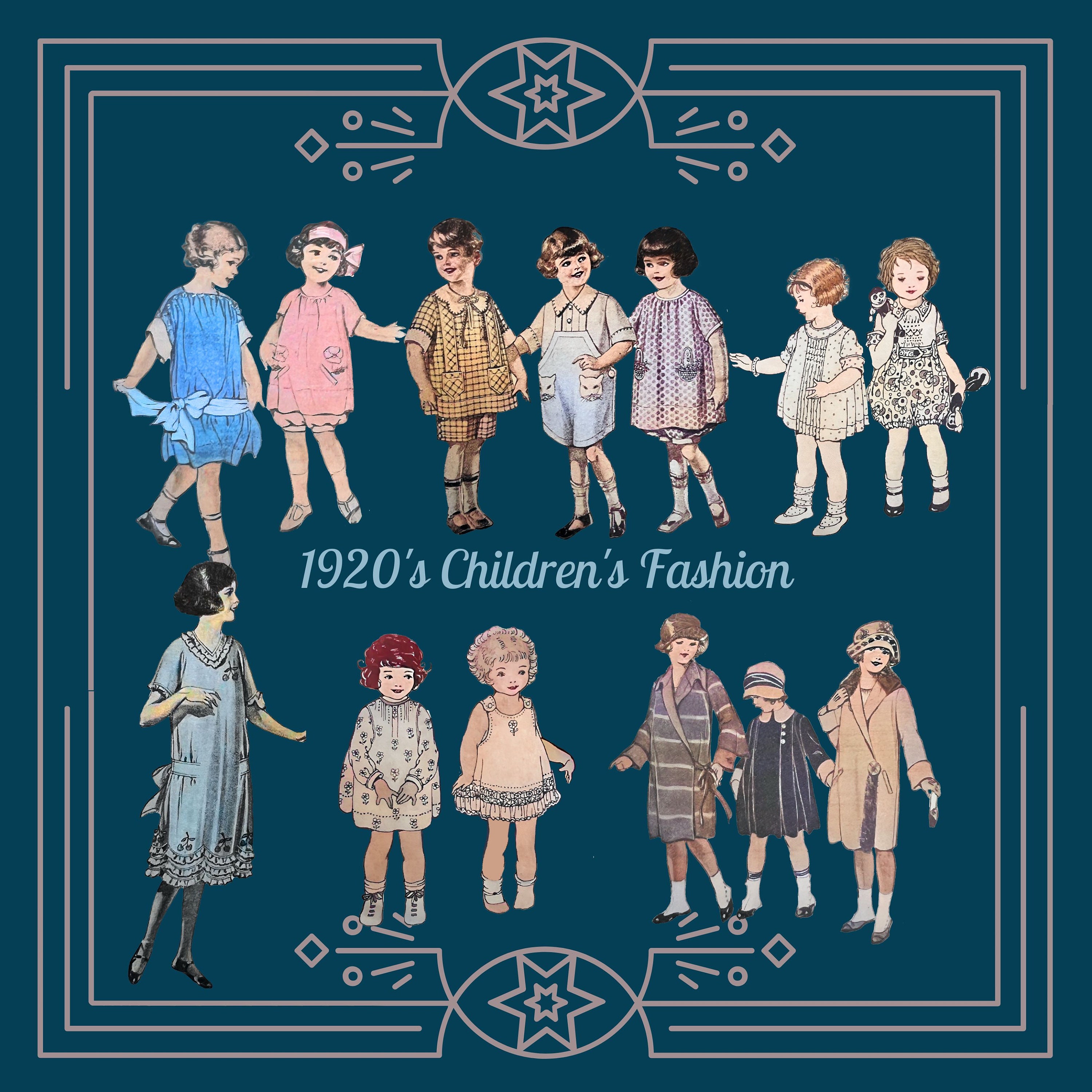The advertisement, titled "1920s Children's Fashion," showcases a vibrant display of period-specific clothing and haircuts. Encased within a distinctive Art Deco frame featuring blue and star-studded patterns, the ad provides a rich visual presentation of fashionable attire for children ranging in age from toddlers to preteens and teenagers. There are drawings of twelve girls and boys adorned in various outfits. The girls sport dresses with bows, some in pink and blue hues, while the boys wear checkered shirts, shorts, and overalls with playful patterns. Each child features appropriate hairstyles from the era, adding to the authenticity of the scene. Off to the side stands a woman, possibly a mother or teacher, wearing a 1920s-style dress with a bob haircut, epitomizing the fashion of the time. This detailed depiction captures the essence of children's clothing and aesthetics from the 1920s, making it a charming and educational piece reflecting historical apparel trends.